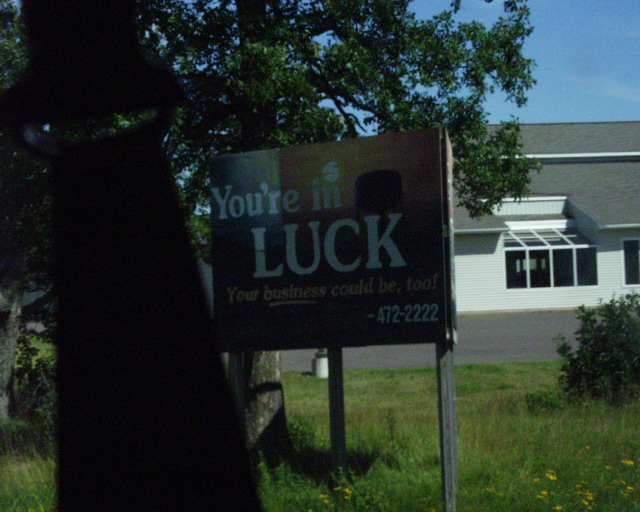In this image, a prominent sign is situated behind a tree with a white house and its driveway visible in the background. On the left-hand side, a vertical object resembling a seatbelt climbs upwards. The foreground features green grass sprinkled with yellow dandelions. The sign, supported by three poles, reads "You're in luck. Your business could be too," along with a contact phone number. The text "You're in luck" is in white, "Your business could be too" is in yellow, and the phone number is in white, all set against a black background. Above the sign is a tree with dark green leaves. The right side of the image showcases the white house with a gray roof and a gray driveway. In the top right corner, the sky is a light blue, completing the scene.